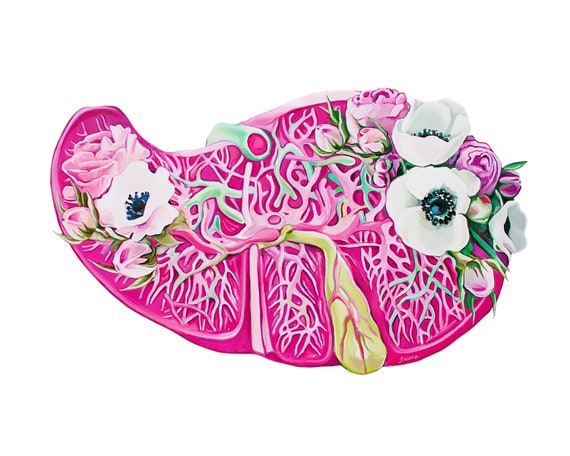The image depicts an intricate, hot pink illustration of a liver or a paisley-shaped organ. The organ is filled with a network of vein-like lines that vary in shades of light pink, with some featuring white tips and light green segments. To enhance the allure of the artwork, the organ includes a few floral elements. Clusters of flowers are situated at both the wider, rounded part on the right, and more narrowly curved side on the left. These flowers, which include white poppies with dark blue centers and pink roses surrounded by green leaves, add a whimsical touch to the otherwise anatomical depiction. Additionally, there's a prominent turquoise duct at the top and a yellowish duct or sac near the center-bottom. All of this is set against a stark white background, highlighting the vibrant, detailed nature of the illustration.